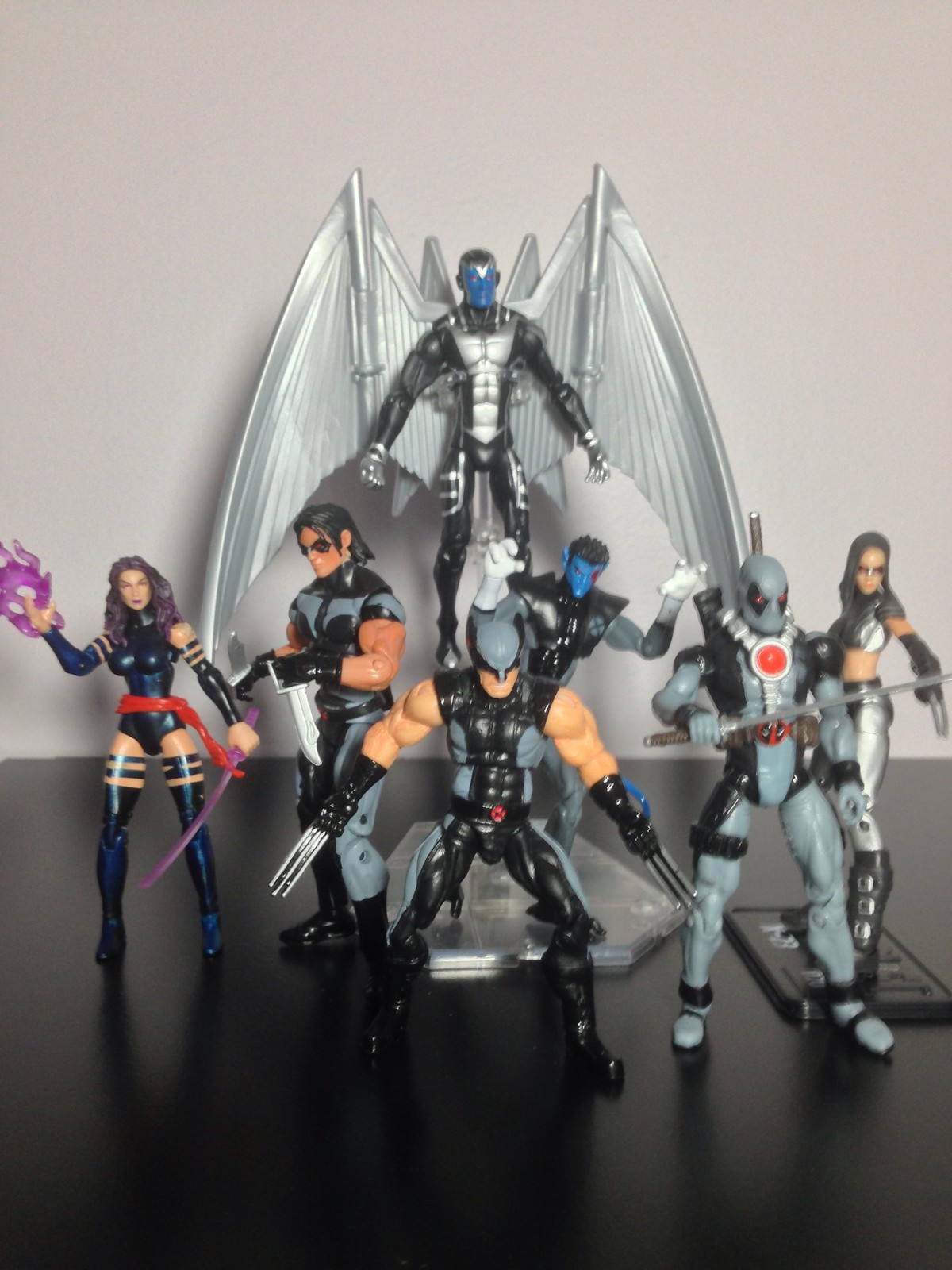This indoor image, likely taken in a child's bedroom, displays a group of seven detailed comic superhero figurines placed on a black table or countertop against a solid white wall. The central figurine is Wolverine, characterized by his tan arms, black and gray outfit, and signature metal claws protruding from his gloves. To Wolverine’s right stands Deadpool, also dressed in a black and gray costume, wielding two plastic knives. In the back, a floating figurine with silver wings adds a dynamic touch to the scene. Among the group are two female superheroes; one brandishes a purple sword in her left hand and has an ethereal purple flame in her right, while the other features metal claws coming out of her hands. The arrangement is centralized in the frame, highlighting the vibrant color palette of black, gray, blue, purple, red, and silver amidst the otherwise monochromatic room setting.